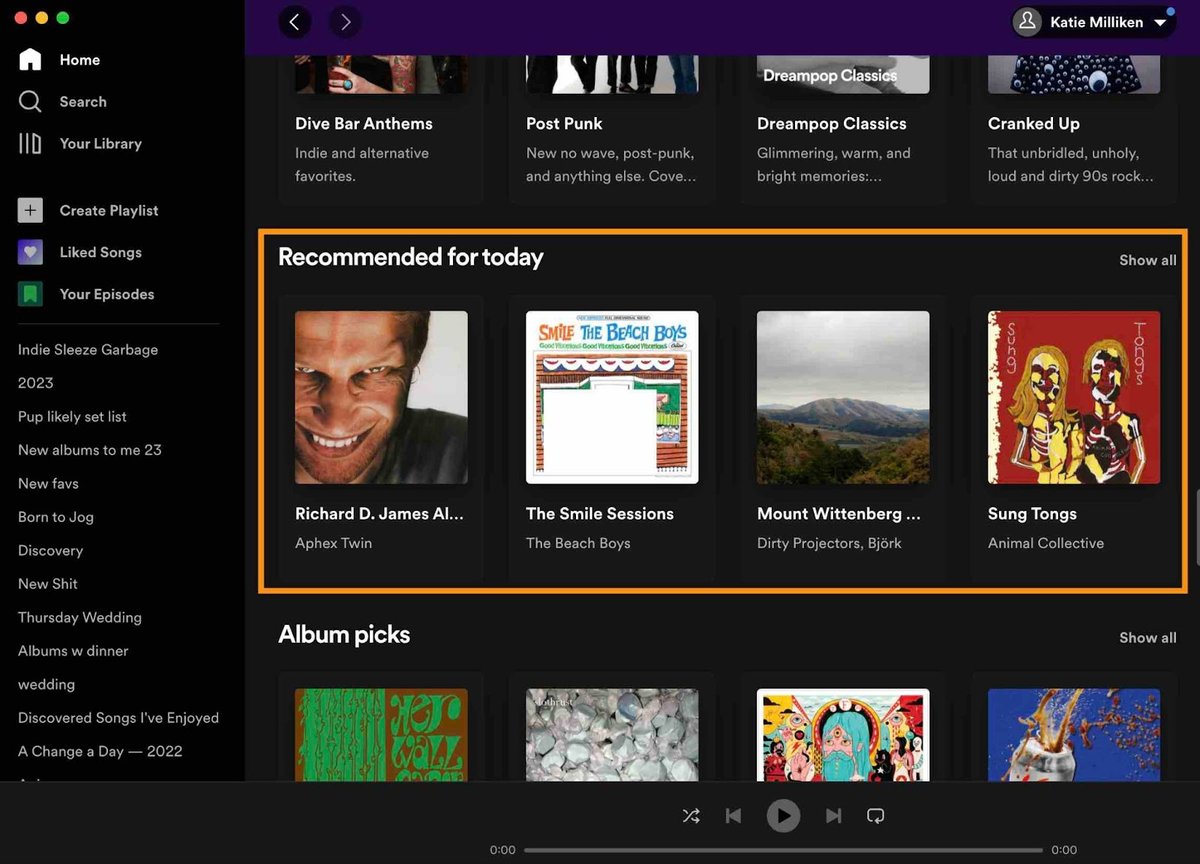The image is a detailed screenshot of the Spotify application on a computer, showcasing its dark-themed, predominantly black interface with vibrant pops of color from various album covers. On the left, there's a navigation panel listing options such as Home, Search, Your Library, Create a Playlist, Liked Songs, and Your Episodes. Underneath these options, an expansive list of personalized categories is visible, including Indie, Sleaze, Garbage, 2023, Pup, Likely, Set List, New Albums, To Me, 23, New Faves, Born to Jog, Discovery, New Shit, Apologies for that, Thursday, Wedding, Albums with Dinner, Wedding, Discover Songs I Have Enjoyed, A Change of Day, and 2022.

At the top of this sidebar, a purple bar displays an account-related section with bi-directional arrows and an account name, Katie McKillen, alongside a Dropbox icon. 

The main area of the app displays several music recommendations. Featured prominently are categories like Dive Bar Albums, Post Punk, Dream Pop Classics, and Cranked Up. An orange-highlighted box below these sections signals today’s music recommendations, listing albums such as "Richard D. James" by Aphex Twin, "Smile Sessions" by The Beach Boys, "Mount Wittenberg Orca" by Dirty Projectors & Björk, and "Sung Tongs" by Animal Collective.

Towards the bottom, a partially visible section titled "Album Picks" appears with a 'Show All' option, hinting at additional selections. Below the album displays, the playback control bar is faintly visible, featuring essential controls for play, pause, and skipping tracks.